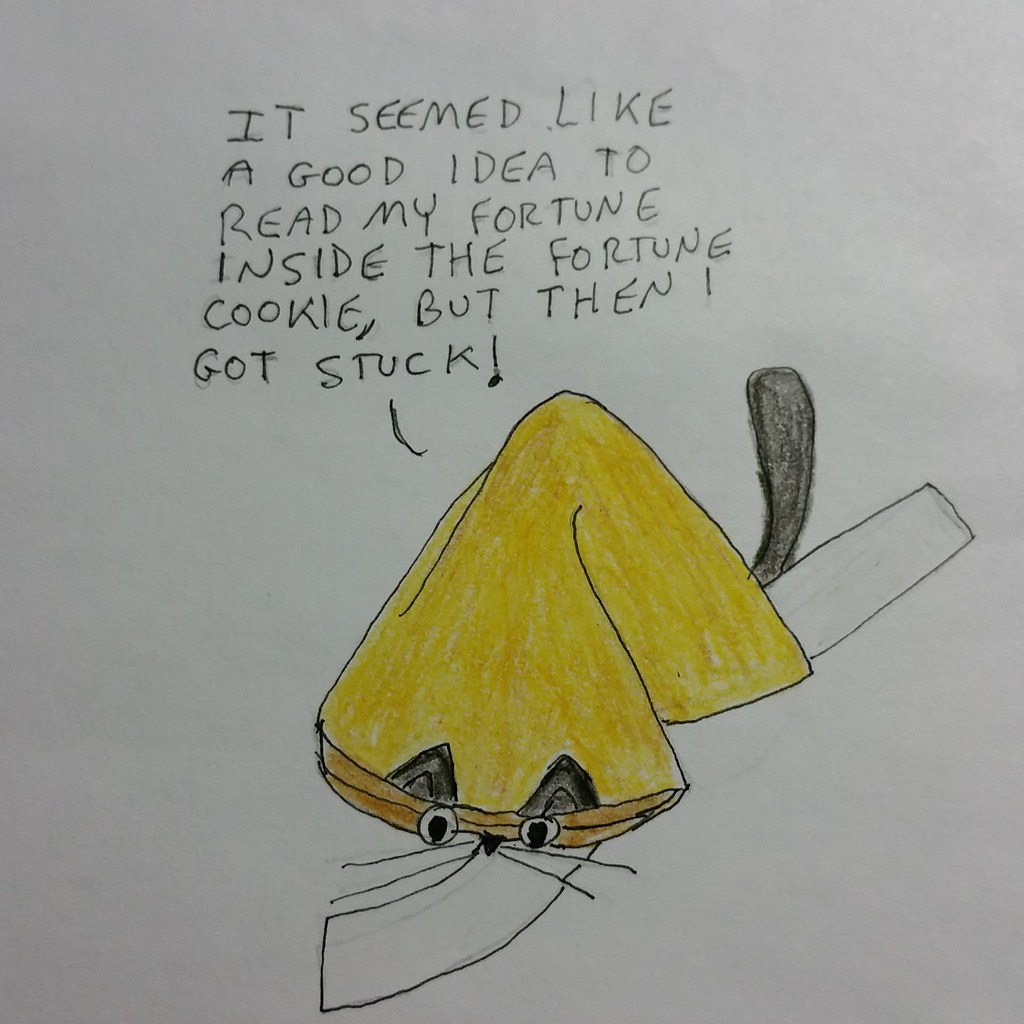The image features a cartoon-style drawing on a piece of paper, showcasing a whimsical yellow and orange fortune cookie adorned with detailed cat features, including pointy ears, eyes, a nose, whiskers, and a black tail. The fortune cookie is sealed shut with a fortune paper humorously protruding from both ends. Above the drawing, handwritten in black text, is the caption: "It seemed like a good idea to read my fortune inside the fortune cookie, but then I got stuck!" The background is plain and off-white, keeping the focus on the playful, hand-drawn illustration of the feline fortune cookie situation.